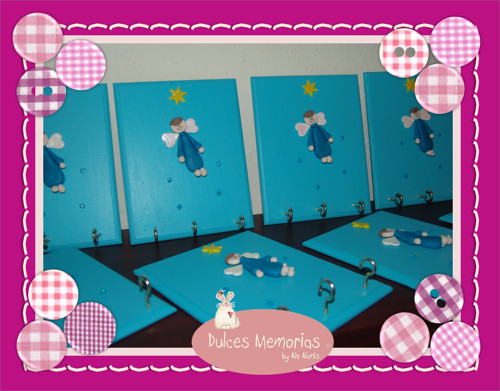The image features a digitally framed photograph showcasing handcrafted wall panels. The frame is a bright purple, with intricate white lacing patterns near the inner edges, giving it the appearance of a postcard. Each corner houses three decorative buttons with a checkered pattern consisting of pink and white squares, with some buttons featuring dots. At the bottom of the frame is a pink oval with blue-white text reading "Dulce Memorias," although part of the text is obscured. In the center of the frame is a rotund, white cartoon bunny with small ears and a round body. 

The focus of the photo is on the small rectangular wooden panels painted light blue, each featuring three small silver eye hooks along the bottom edge. Each panel has a slightly cartoonish woodcut angel with pure white skin, adorned in a blue dress and sporting delicate wings, under a yellow six-point star. There are four such panels positioned upright against a white wall in the background, and another four lying flat on a black table surface in the foreground. The scene appears to have been crafted for a website or promotional material, with the text suggesting its Spanish origins.